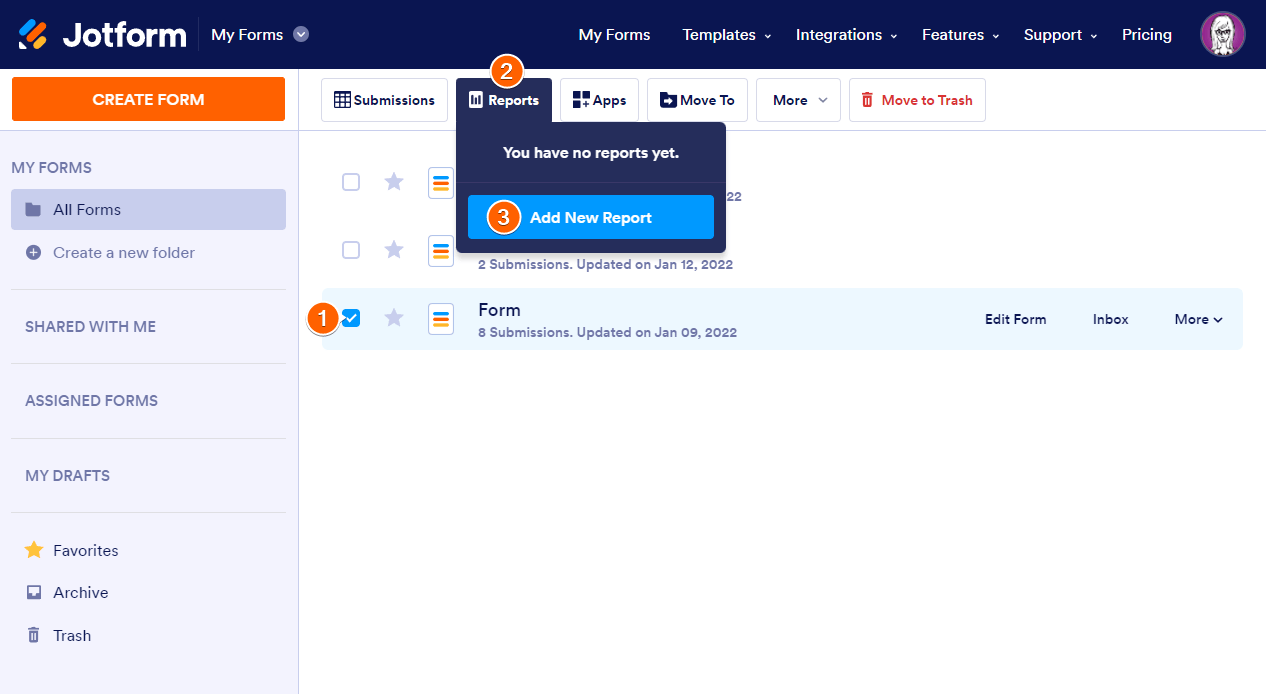Here is a detailed and cleaned-up description for the screenshot:

---

A screenshot of a website interface, likely representing a form creation and management platform. The top of the webpage features a black background with predominantly white text. On the left side, there is a colorful logo comprised of blue, red, and green elements. Next to the logo, the text "Job Form" is displayed in white, followed by the tagline “This is my form.”

To the right, the navigation menu contains links labeled "My Forms," "Templates," "Integrations," "Features," "Support," and "Pricing," alongside an avatar icon—a photograph of a person set within a blue circle outlined in white.

On the left side beneath the header is an orange button with the white text "Create Form." Below this, a vertical navigation menu is seen in a grey box with bluish text. The text alternates between blue and gray, with the options reading: "My Forms" (highlighted in blue), "Create a New Folder," "Shared with Me," "Assigned Forms," "My Drafts," and at the bottom, a yellow star preceding "My Favorites," followed by "Archives," and "Trash."

On the right side of the screen within the broader white interface, "Submissions" and "Reports" are sections displayed. The "Reports" section is highlighted in blue, with a message that reads "You have no reports yet" in white text. There is also an icon indicating two notifications, marked with a yellow or orange circle above the "Reports" section.

Below these sections, additional options include "Apps," "Move To," "More," and "Move To Trash." The main content area shows three forms listed, with one form at the bottom highlighted. This form is marked with a blue checkmark and labeled "Form 8 submissions, updated Jan 09, 2022."

---

This refined caption provides a clear, structured, and detailed overview of the depicted website interface.